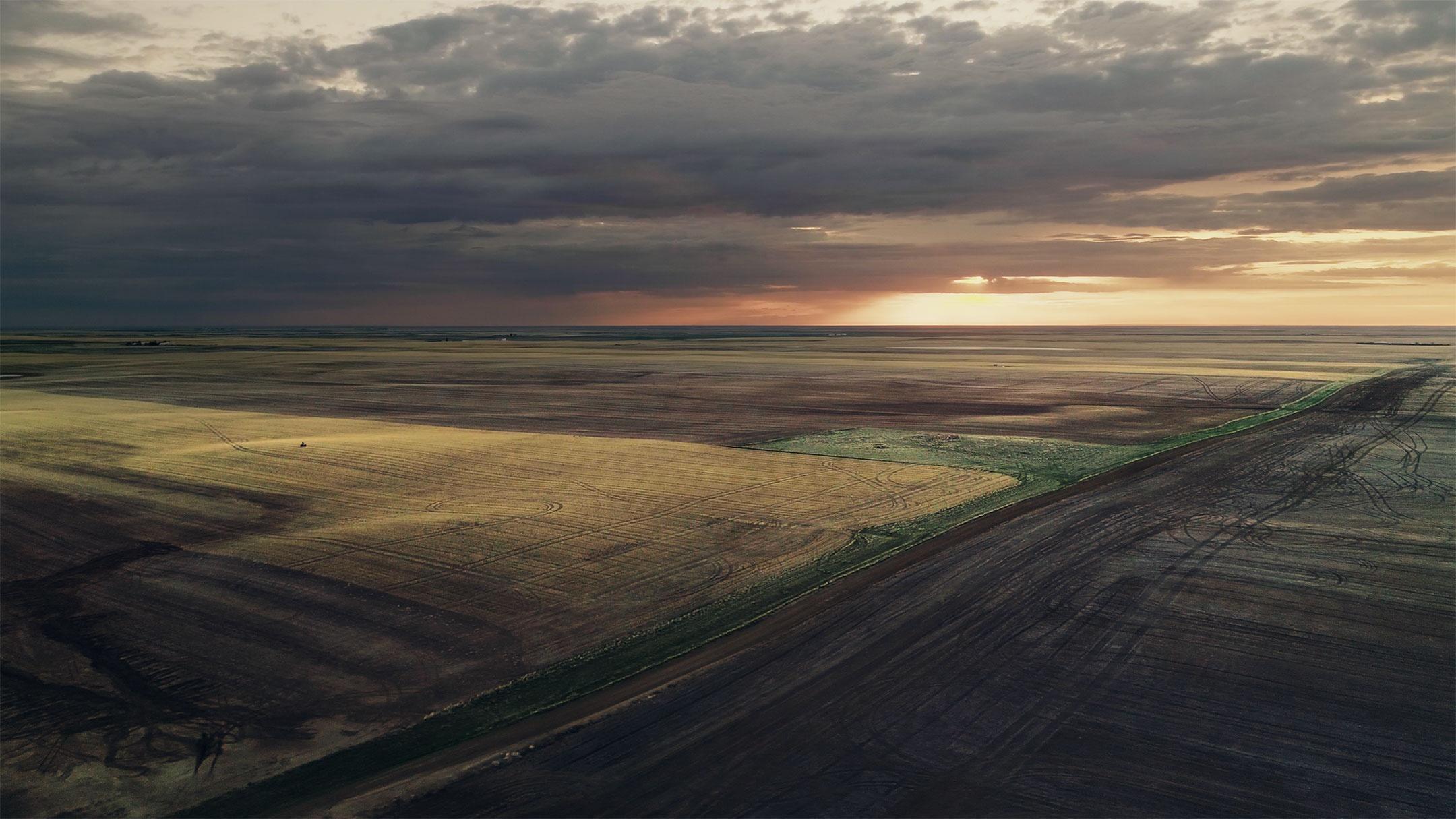This aerial color photograph, taken from a drone or airplane, showcases an expansive landscape of agricultural plains stretching for miles. The fields are a patchwork of colors and textures: golden wheat fields, green fields, and freshly tilled brown fields etched with tractor tracks. A single-lane dirt road slices through the middle of the image, separating a vibrant wheat field on the left from a freshly tilled plot on the right. The photograph is oriented horizontally, with the plains occupying the bottom half of the image, giving way to a dramatic sky above. The setting sun creates a gradient of colors from yellow and gold at the horizon to deep reds and oranges, gradually darkening to reveal black rain clouds that loom overhead. This blend of colors and natural patterns highlights the beauty and complexity of rural farmland in a real-world, representational style.